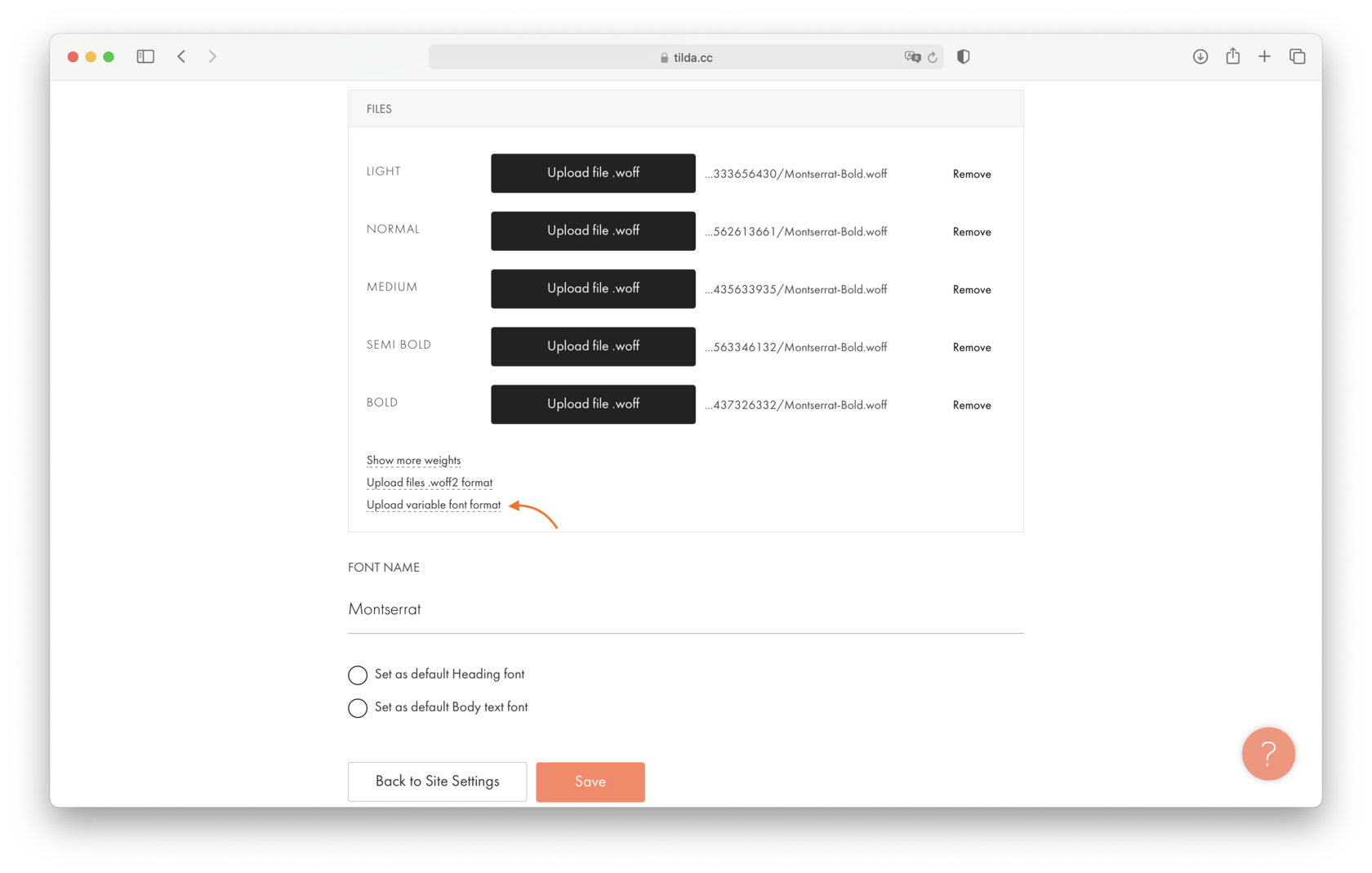Here's a descriptive and detailed caption based on the provided voice note:

---

This screenshot captures a web page viewed on an Apple desktop, identified by the signature gray bezel at the top that includes a red circle, orange circle, and green circle, which are standard for Apple interface. The top bar also features a square with a smaller rectangle inside it, alongside a black arrow pointing left, indicating a back function, and a gray, non-functional forward arrow. 

Below this, a dark gray, rounded URL search bar displays a gray lock icon to its left and the web page address "TILDA.CC" in black text. Adjacent to this, there are icons: a square with an "A", a square with an "S" featuring a black background and a white "S", followed by a circular refresh symbol composed of two arrows forming a circle. A shield icon, split into black and white halves, is next, followed by a circle with a down arrow for downloads, a square with an up arrow for uploads, and a plus icon to open new windows. Further along, two overlapping squares signify the ability to manage multiple open windows.

The primary content area is a large white rectangle with a gray header labeled "Files" on the left. Within this space, there are rectangles labeled "Upload File.WOFF", each associated with different font weights such as Light, Normal, Medium, Semi-Bold, and Bold. Each entry has a "Remove" option and includes a URL to the right. A red arrow points to the bottom section, highlighting the link "Show More Weights", with a note directing to "Size Black". Additionally, there's a section labeled "Upload Files.WOLF2 Format" and another for "Upload Variable Font Format."

Outside this main rectangle, the page has a highlighted section for font settings. "Font Name" is written in all capital letters with "M-O-N-T-S-E-R-R-A-T" directly below. Two selectable circles follow, one labeled "Set as Default Heading Font" and the other "Set as Default Body Text Font". At the bottom, there are two buttons: a white one with black text labeled "Back to Site Settings" and an orange/off-orange one labeled "Save." Finally, on the far right, there is a circular icon with a white question mark in the same off-orange color scheme.

---

This detailed caption describes the visual elements, layout, and functionality present in the screenshot comprehensively.